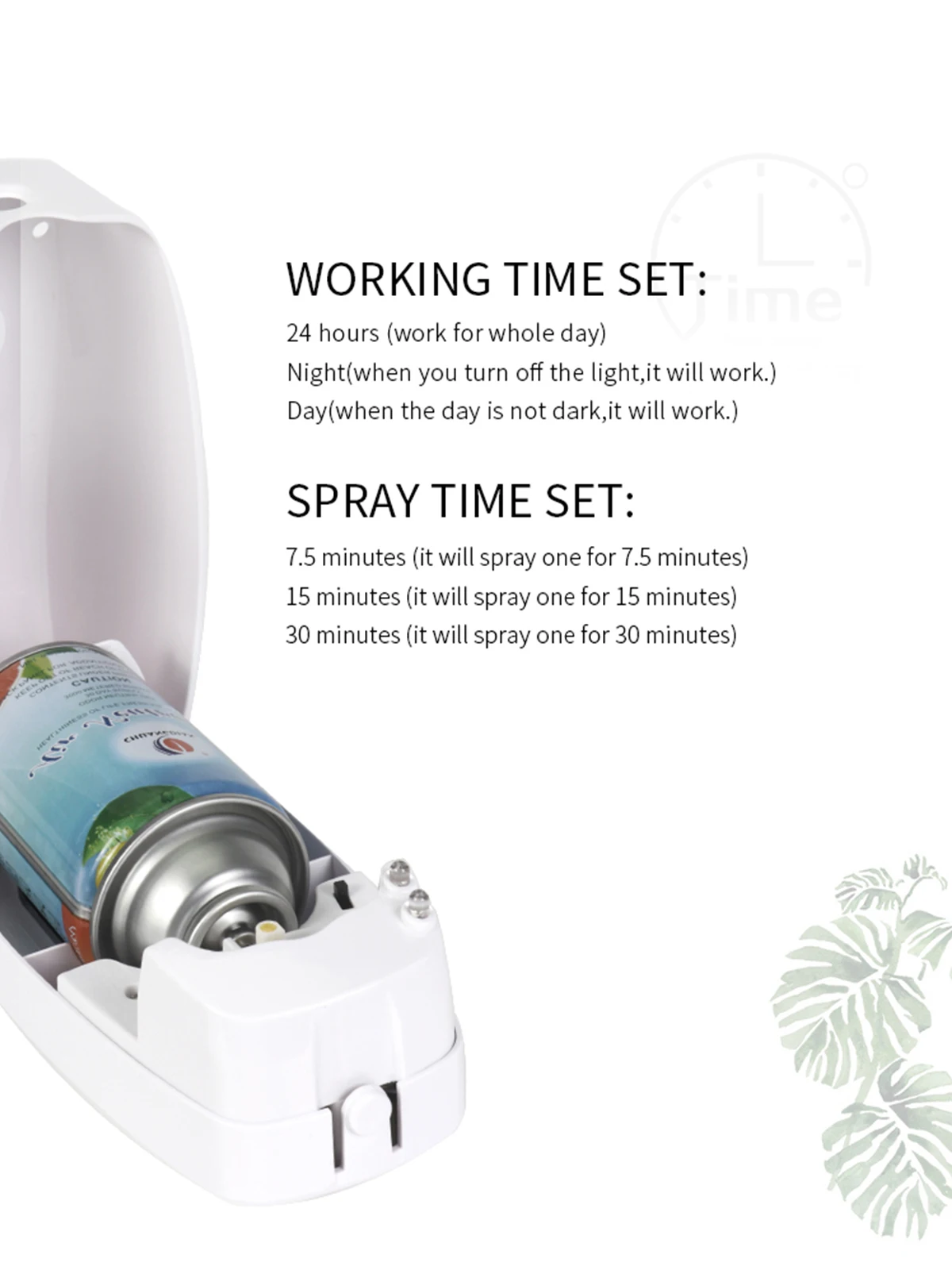The photograph features an automatic aerosol dispenser unit, typically used for releasing pleasant scents into the air. The unit, which is white, is opened on the left side, revealing an aerosol canister inside. The canister has a light blue label adorned with a green leaf design and some central text, although the label is facing away from us. On the right side of the dispenser, there are two indicator lights and a black switch likely for turning the unit on or off. The background of the image is white, with a subtle, light green leaf print in the bottom right corner. The center of the image contains black text detailing the operational settings: "Working time set 24 hours – works for a whole day. Night: when you turn off the light, it will work. Day: when the day is not dark, it will work." Below that, the text continues: "Spray time set: 7.5 minutes – it will spray once every 7.5 minutes; 15 minutes – it will spray once every 15 minutes; 30 minutes – it will spray once every 30 minutes." This description provides a comprehensive view of the product and its functionality, emphasizing both the visual and textual elements present in the photograph.